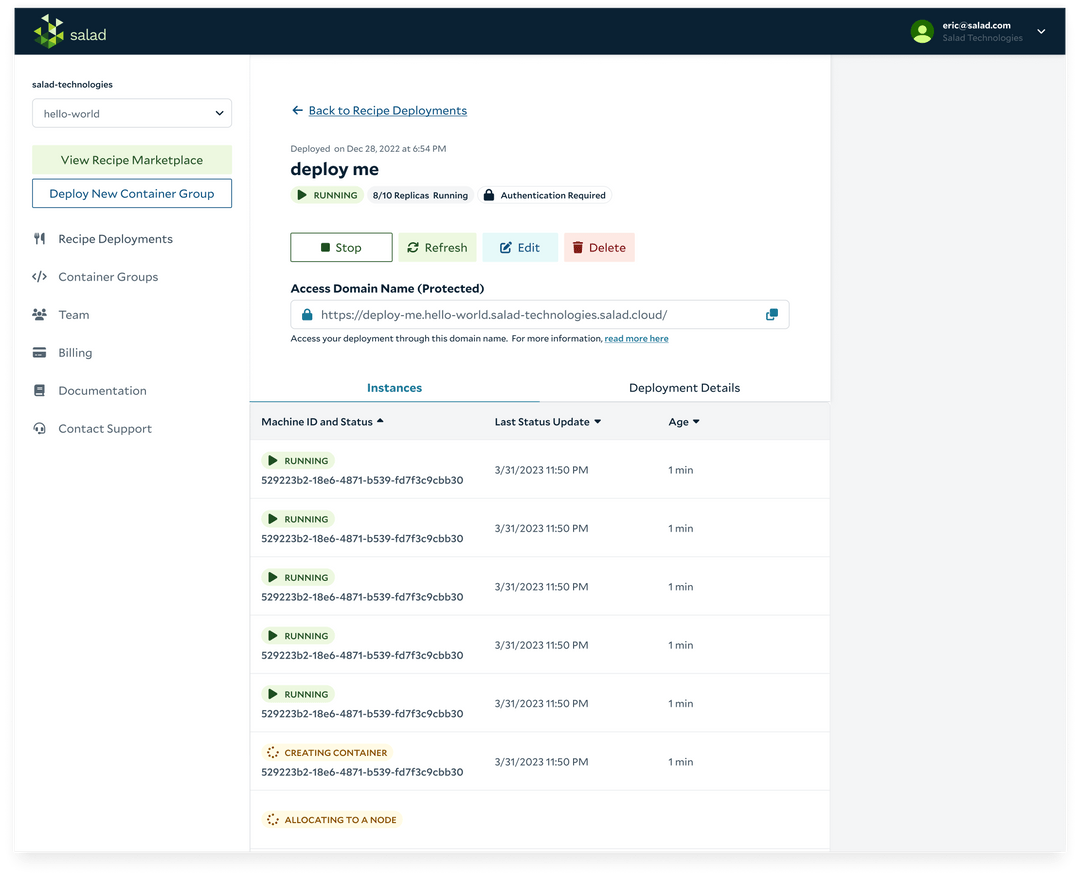The image captures a section of a website with a primary focus on a platform for managing container deployments. Here is a detailed caption:

---

The image is a screenshot from a website focusing on container management. At the top, a thin black bar spans the width of the page, containing a green word "Salad" followed by an abstract square composed of various shades of green. On the right side of the bar, there's a small cartoon icon of a person in a green circle, next to a blurred email address in white text. A down arrow further suggests a drop-down menu feature.

Below this top bar, the screen continues with a clean white background and predominantly black text displaying "Salad Technologies." Adjacent to this title is a pull-down menu highlighted in white. Below, there are two main action buttons: a green box labeled "View Recipe Marketplace" and a blue box labeled "Deploy New Container Group."

The subsequent section features a navigation sidebar in gray displaying various options: "Recipe Deployments" (with a knife and fork icon), "Container Groups" (with arrows icon), "Team" (depicted by small cartoon people), "Billing" (credit card icon), "Documentation" (book icon), and "Contact Support" (headset icon).

Further down, a blue header states "Back to Recipe Deployments." Below it, in gray text, appears the deployment information: "Deployed on December 28th, 2022, at 6:54 PM." 

This is followed by several status indicators: a green box reading "Running," alongside gray boxes indicating that 8 out of 10 replicas are running, and another gray box with a padlock icon reading "Authentication Required." 

Additional action buttons are found next: "Stop" (green), "Refresh" (green), "Edit" (blue), and "Delete" (red).

Further along, it mentions the domain access status: "Domain name protected" with a blue padlock icon next to the protected domain name. Instructions follow: "Access your deployment through this domain name for more information read more here."

Below this section, a blue header labeled "Instances" lists machine IDs and their statuses, with most showing "Running" (indicated by green text). One instance is marked "Creating Container" in orange, and another as "Allocating to a node." Each instance includes a last status update of "March 31st, 2023," and an age indicator noting "1 minute."

---